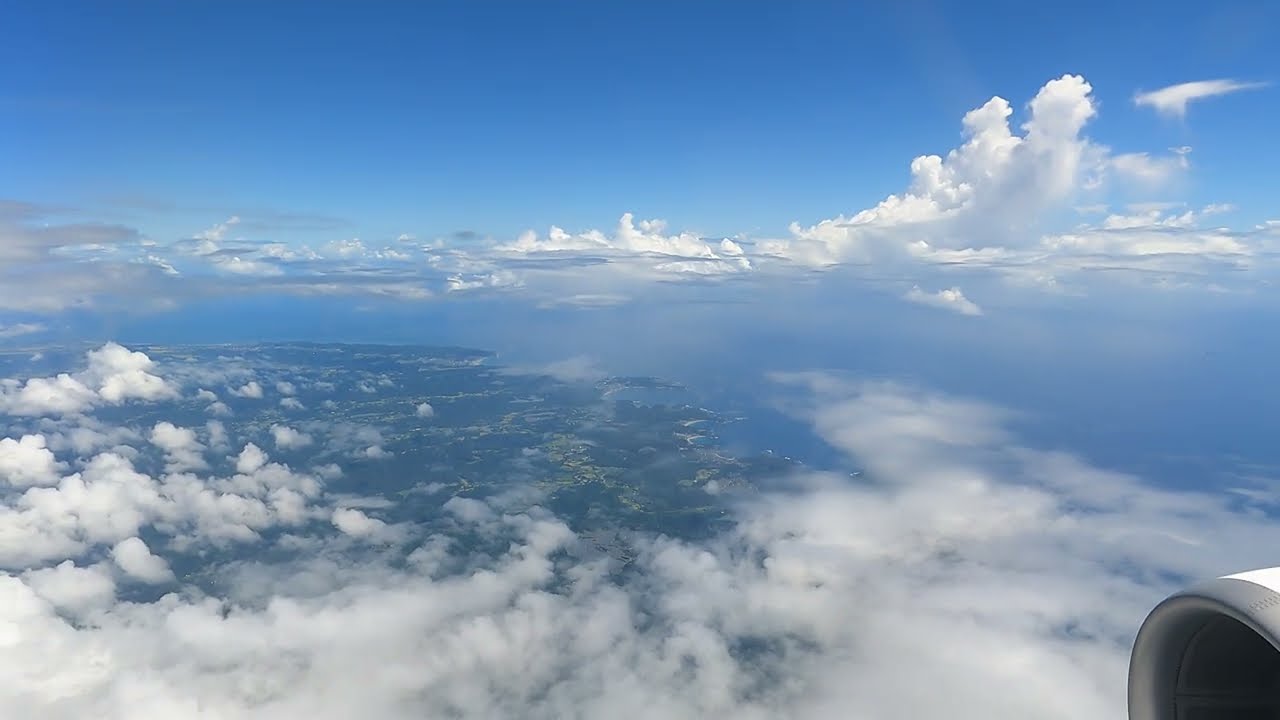This captivating photograph, taken from inside an airplane, offers a mesmerizing aerial view. A white airplane engine with a silver rim is prominently featured in the bottom right-hand corner. The viewer's eye is drawn to the stunning juxtaposition of fluffy, white clouds both close by and in the distant background; the cumulus clouds in the top right add depth to the scene. Below, the land stretches from the bottom left toward the middle, revealing patches of green vegetation, dirt, and indistinct buildings. This diverse terrain meets the vast ocean, which gracefully blends into the serene blue expanse of the sky. The image beautifully captures the essence of high-altitude travel, highlighting the harmonious convergence of earth, water, and sky.